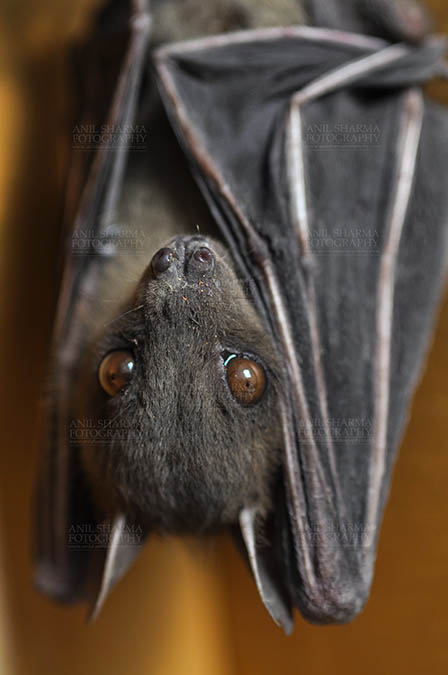In this detailed color photograph, a young, furry bat is pictured hanging upside down in a portrait orientation. The bat, which exhibits a grayish-brown hue, has short hair and a pointed, triangular-shaped nose. Its face is predominantly black, accented by two beady brown eyes and small nostrils. The bat's long, tapered ears point downwards. Its wings are closed near its body, featuring a dark gray membrane with a light gray bony structure creating a web-like pattern. The background showcases a golden brown color, giving the impression of drapery, which emphasizes the bat as the main subject. Captured by Annie Shamira Photography, the bat appears alert and engaged, peering out at the viewer from its inverted position.